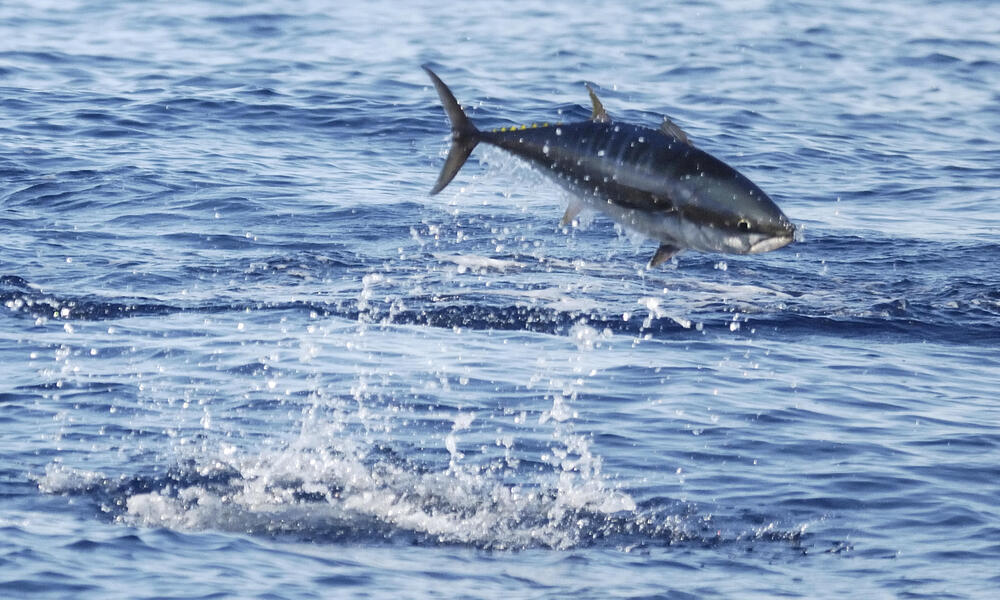This captivating photograph captures a single fish, likely a type of tuna, in mid-leap above a sprawling blue expanse of calm ocean water. The action shot, taken horizontally, features the fish jumping towards the right side of the frame, creating a dynamic sense of motion. The fish, displaying shades of bluish-black and gray with a silver belly, glistens under the sunlight, emphasizing the detailed textures of its scales. Its one visible eye and mouth are clearly discernible, hinting at its path and vigor.

Beneath the airborne fish, a prominent splash can be seen where it broke the surface, sending white, foamy water droplets scattering in all directions. The surrounding water remains relatively calm, with gentle ripples spreading outward, colored in various shades of blue reflecting different depths and shadows. The serene, nearly glassy waters provide a stark contrast to the burst of energy at the splash point, making the fish's leap the focal point of the image. This vivid composition showcases the harmony and contrast of a solitary ocean scene.